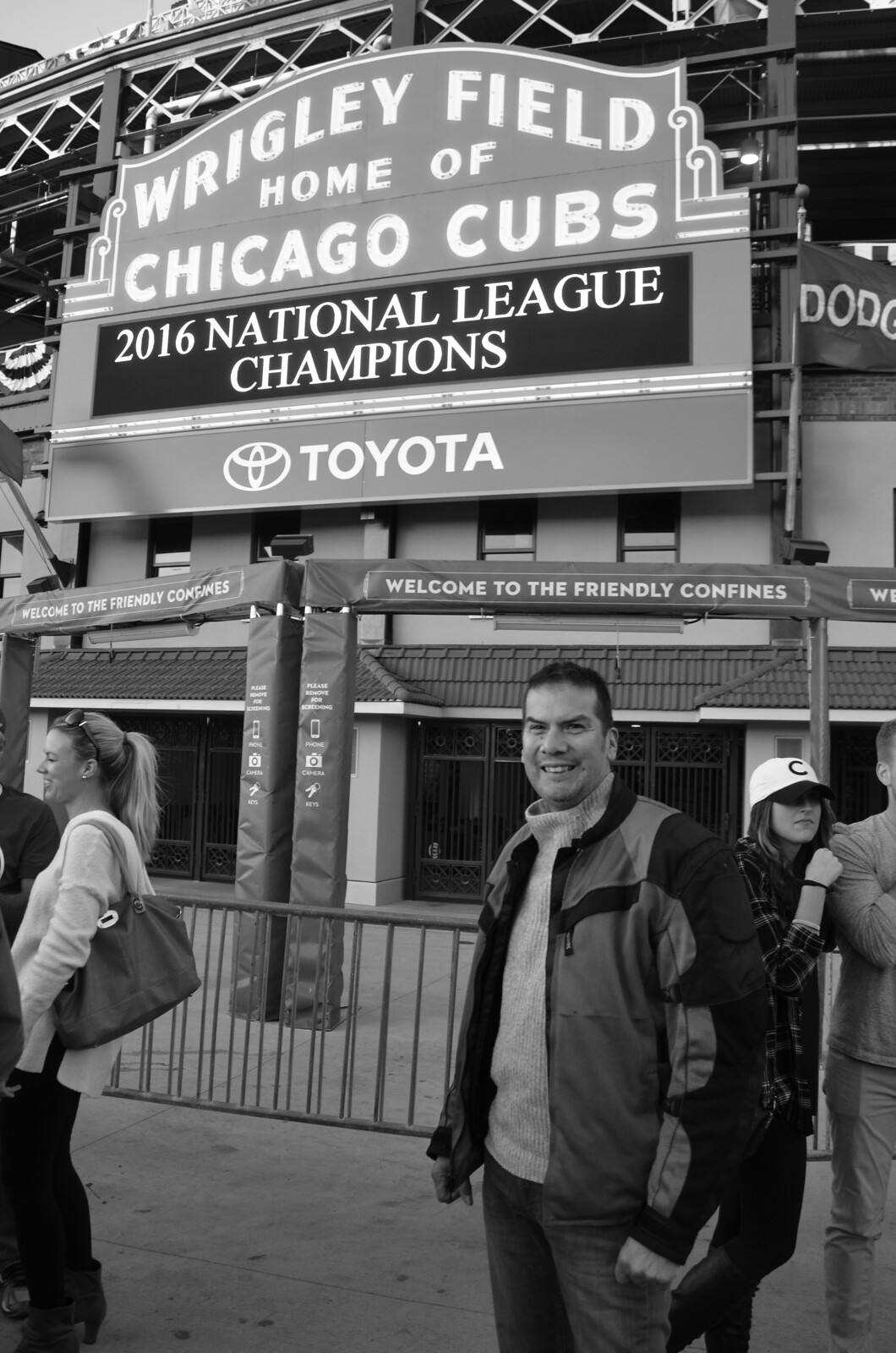In this modern black and white photograph, a man with short hair, wearing a sweatshirt, jacket, and jeans, poses with a big smile on his face. The image, likely taken on a smartphone, is noticeably taller than it is wide, suggesting a casual, amateur snapshot. He stands in front of the iconic entrance to Wrigley Field, home of the Chicago Cubs, which is adorned with a prominent sign that reads, "Wrigley Field, home of Chicago Cubs." Beneath that, a digital display proudly states, "2016 National League Champions," alongside a Toyota logo and the welcoming phrase, "Welcome to the Friendly Confines." Surrounding the man are various people, including a woman wearing a Chicago Cubs hat, who appears to be exiting through the gated area of the stadium, indicating the lively atmosphere outside the ballpark.